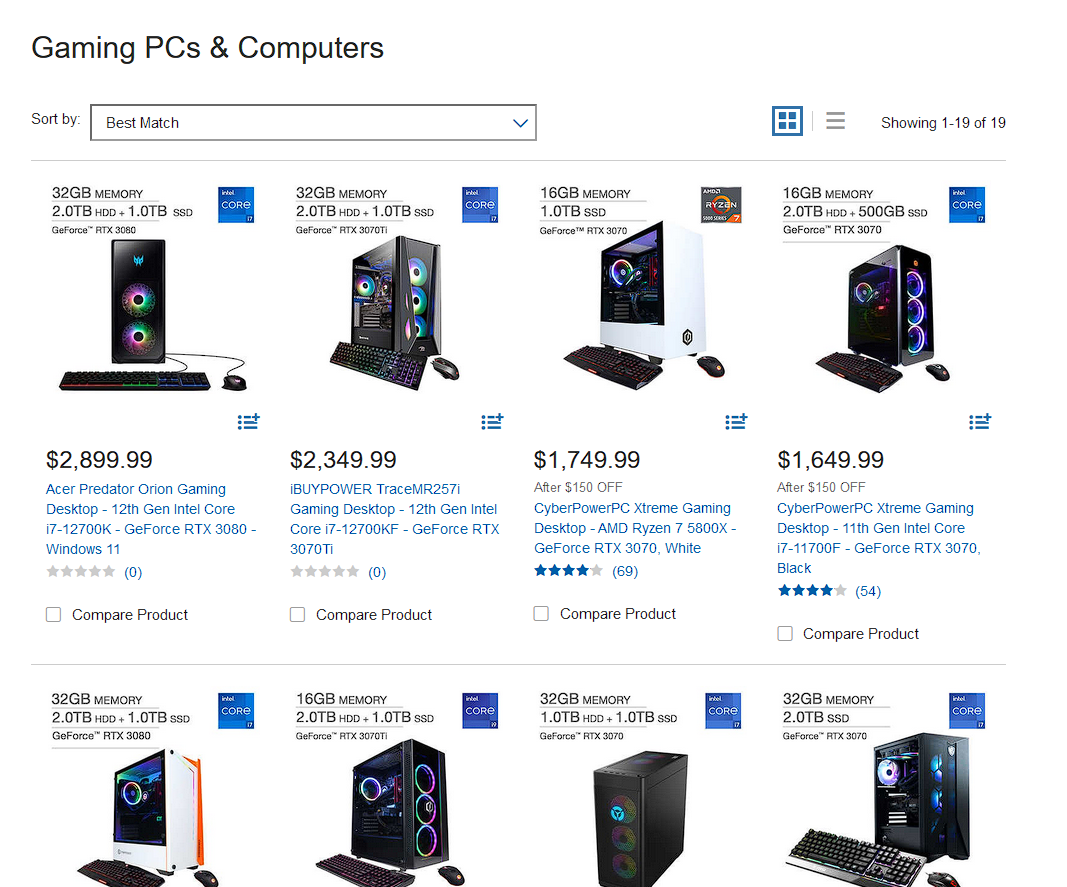The image depicts a web page interface for an online store that sells games, PCs, and computers. The layout is roughly square, with an undefined edge due to the white background. In the upper left corner, black text reads "Games, PCs, and Computers." Below this, on the left, there is a "Sort by:" label followed by a search bar with a dropdown menu currently set to "Best Match" in blue text.

To the right of the search bar, a blue icon with four squares allows users to change the listing display format, accompanied by a gray icon with three horizontal lines for the main menu. Further to the right, text indicates "Showing 1 through 19 of 19."

Below, the page displays a grid of desktop computer tower images, arranged in four columns and two rows, making up a total of eight visible items. These towers feature multi-colored, rainbow-like fans. The prices for the visible computers range from $1,649.99 to nearly $2,900, although the prices for the bottom row are not fully visible.